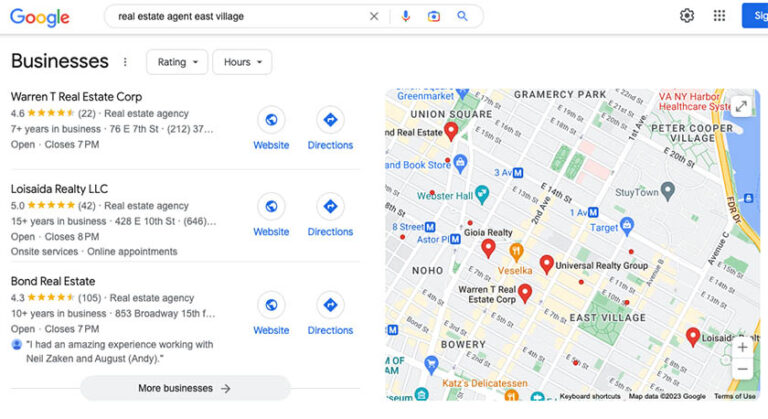Screenshot of a Google search for "Real Estate Agent East Village," displaying the top three results. The search bar with the Google logo is positioned at the top. Below, three different real estate businesses are listed:

1. **Warranty Real Estate Corp**: Rated 4.6 out of 5 stars based on 22 reviews, with links to the website and directions.
2. **Loiseta Realty LLC**: Rated 5 out of 5 stars from 42 reviews, also with links to the website and directions.
3. **Bond Real Estate**: Rated 4.3 out of 5 stars with 105 reviews. It includes a portion of a review stating, "I had an amazing experience working with Neil Zakin and August (Andy)." Links to the website and directions are also provided.

On the right side of the search results, a map of East Village highlights the locations of these businesses with red icons. Several other businesses are marked on the map, and it is interactive, allowing movement to explore additional search results in the area.